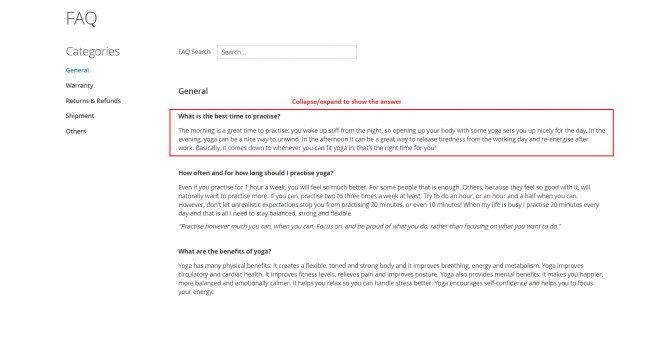This is a detailed caption for the image:

"The image is a screenshot taken from a Google FAQ page pertaining to Microsoft. The highlighted section of the screenshot shows a question in bold text that reads, 'What is the best time to practice yoga, and how often and for how long should I practice yoga? What are the benefits of yoga?' The first question is enclosed within a red rectangle and includes added text indicating 'collapse/expand to show the answer.' Below this query, the page lists several categories for further information: 'General,' 'Warranty,' 'Returns and Refunds,' 'Shipment,' and 'Others.' The screenshot provides insight into a wealth of information available on the FAQ page, specifically about the practice and benefits of yoga. It emphasizes that even modest engagement, like one hour per week, can significantly enhance health. The design and layout of the webpage suggest a structured and accessible format for users seeking guidance on various topics related to yoga and more."